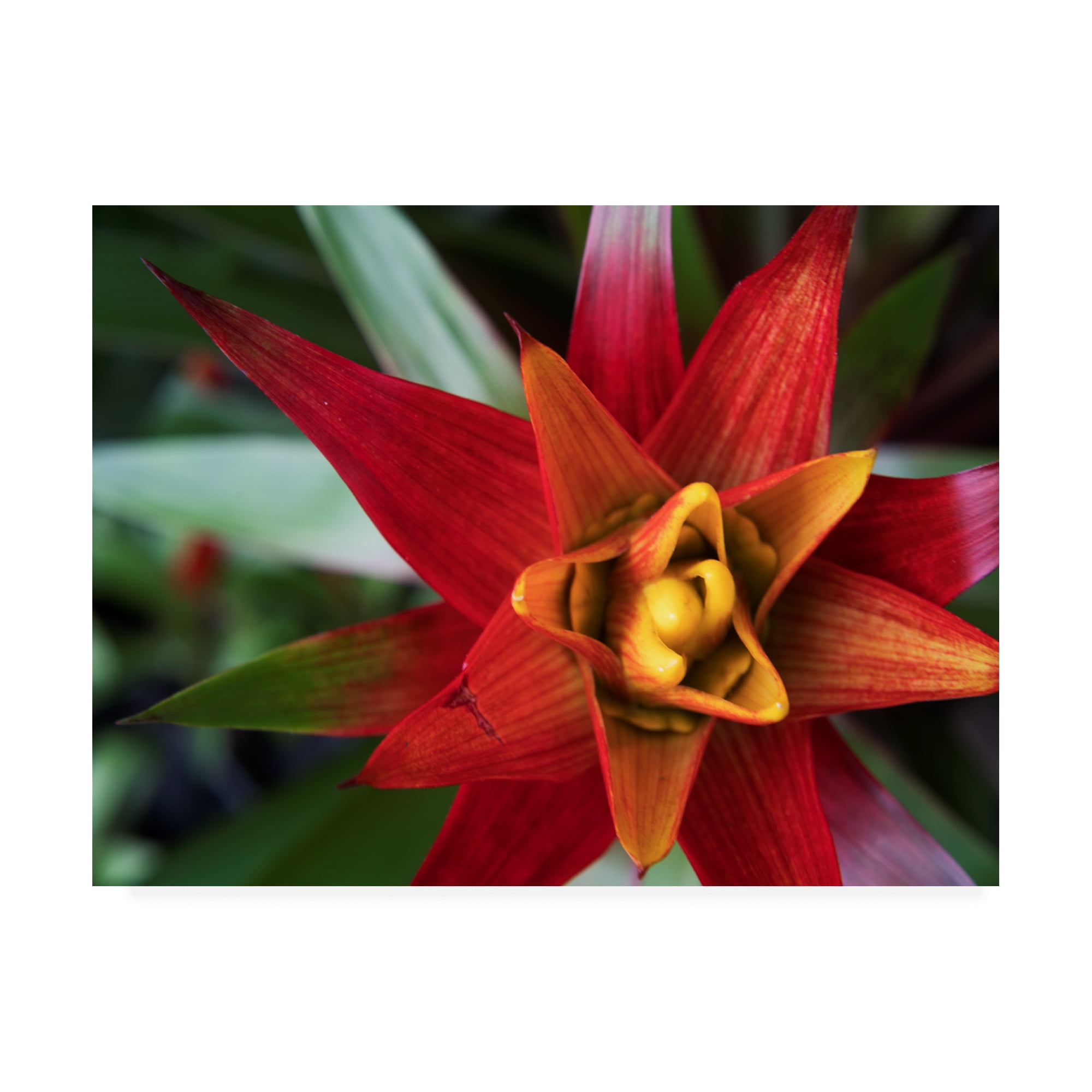This close-up photograph features a stunning red flower with a striking yellow center. The flower nearly fills the frame, positioned slightly off-center to the right, and its petals exhibit a rich gradient of colors—from orangish-red to a deep, blood-red hue. The leaves at the base of the flower are green, contrasting beautifully with the vibrant petals. In the blurred background, more red and green floral elements are vaguely visible, enhancing the focus on the central bloom. The flower's inner structure includes multiple layers or "stars" stacked on top of each other, giving a sense of depth and complexity. A single petal has a small cut, adding character to the otherwise immaculate appearance. This bright and captivating image could easily be framed as artwork, capturing the eye with its vivid colors and intricate details.